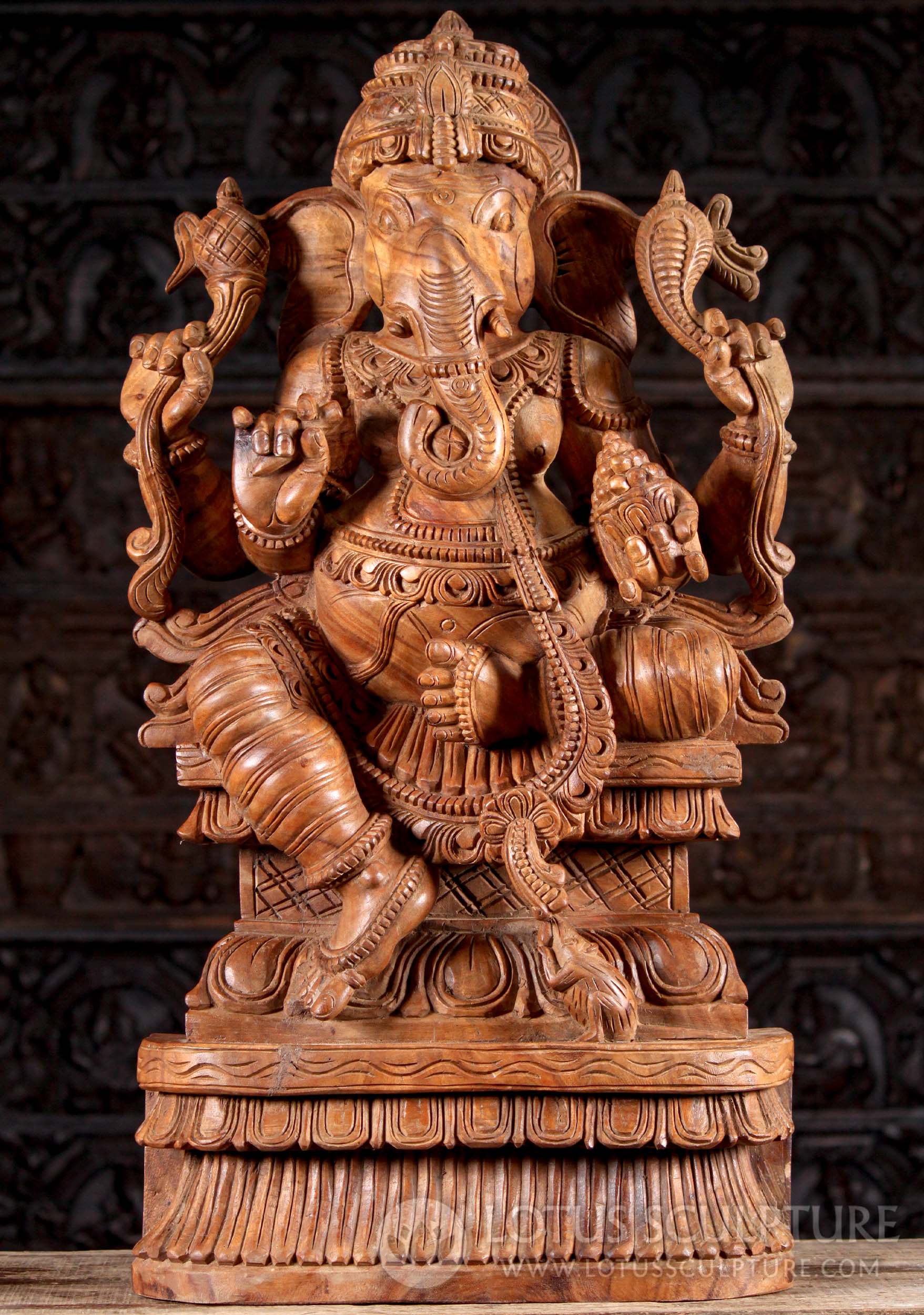The photograph captures a meticulously hand-carved wooden statue, rich in intricate details. The statue depicts a deity characterized by an elephant head and human-like hands, which is emblematic of Hindu iconography, likely representing the Hindu god Ganesha. Ganesha is portrayed in a seated position, with one leg bent and the other hanging off an elaborately carved seat that is integrated into the sculpture. The deity's multiple arms are skillfully detailed, with two top arms holding snakes and others arranged in traditional mudras (symbolic hand gestures). The craftsmanship extends to the elaborate scrollwork and fine details that adorn the statue.

In the background, the image is somewhat dark and blurry but reveals additional carvings and inscriptions that complement the statue, suggesting a religious or cultural significance. The lower portion of the image features a watermark and logo that reads "Lotus Sculpture, www.lotussculpture.com," indicating the source or perhaps the creator of the sculpture. The overall composition highlights the statue's artistry and the cultural richness it embodies.